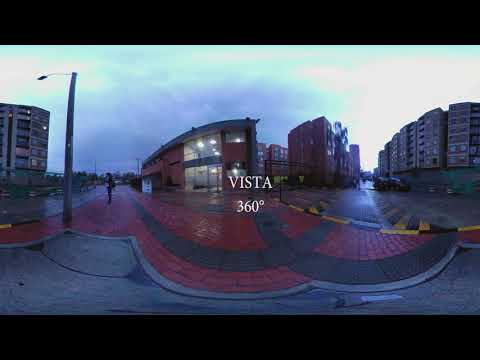The image captures a gloomy evening in a European city, likely Italy, characterized by overcast skies with gray clouds hinting at recent or imminent rain. Central to the scene are several multi-story apartment buildings flanking a red and black patterned brick road adorned with numerous speed bumps. To the left, we observe a seven-story building, while directly in the center background stands a two-story structure with large, open glass windows illuminated by bright white lights. Another series of similar-height buildings, around eight or nine stories high, extend into the right background of the image. The road is lined with streetlights and appears to be wet, further emphasizing the rainy weather. A solitary person, possibly a woman, is seated on the road, and another individual can be seen walking in the image. The bottom and top of the image are bordered in black. Prominently in the center, the text "VISTA 360" suggests a panoramic or wide-angle view of the downtown urban layout. The scene is a blend of architectural simplicity with a somber ambiance, painted in shades of black, white, light blue, dark blue, red, tan, and yellow.